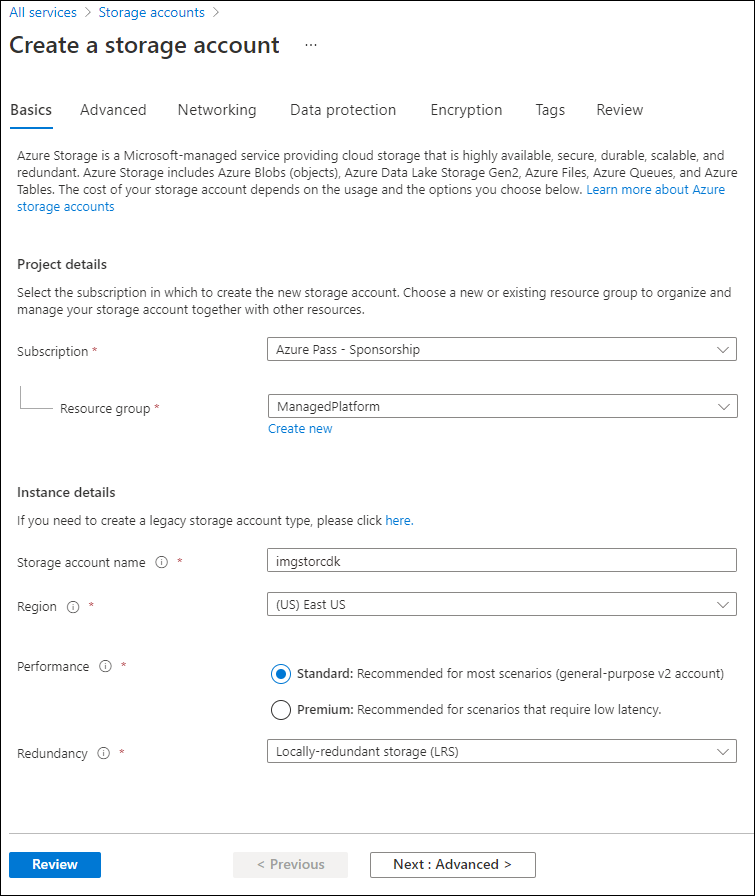The screenshot displays an Azure Storage Account creation form, which is part of Microsoft's cloud storage service. The image is in portrait orientation, resembling an 8.5x11-inch piece of paper. At the very top, the navigation path is indicated in blue text, reading "All services" with a right arrow followed by "Storage accounts" and another right arrow pointing to "Create a storage account."

Below the navigation path, there's a sidebar with different menu options. The currently highlighted option is "Basics," indicated by a blue line underneath it. Other menu options include "Advanced," "Networking," "Data protection," "Encryption," "Tags," and "Review," all displayed in a lighter shade of gray.

The main section of the form provides information about Azure Storage, describing it as a Microsoft-managed service offering highly available, secure, durable, scalable, and redundant cloud storage. It mentions various components like Azure Blobs (objects), Azure Data Lake Storage Gen2, and Azure Files. At the end of this informative paragraph, there is blue text linking to "Learn more about Azure Storage accounts."

Below the informational text, the form is divided into sections:

1. **Project Details**:
   - **Subscription**: Labelled with a red asterisk to indicate a required field, accompanied by a dropdown menu.
   - **Resource Group**: Also marked with a red asterisk and a dropdown menu. There is an option nearby labeled "Create new" in blue text.

2. **Instance Details**:
   - **Storage Account Name**: Followed by a field to input the name.
   - **Region**: Accompanied by a dropdown menu to select a geographical location.
   - **Performance**: Options to choose from, likely via radio buttons.
   - **Redundancy**: Options to select redundancy features, also likely via radio buttons.

At the bottom of the screen, there are navigation buttons for the form. On the left, a blue-filled rectangle with white text says "Review." Next to it, a grayed-out rectangle with the word "Previous" in a lighter gray indicates the backward navigation is disabled. On the right, a white-filled rectangle with black text says "Next: Advanced," followed by a right arrow, suggesting the progression to the next step in the form.

This comprehensive layout helps users systematically create a new Azure Storage account by following the step-by-step instructions provided.